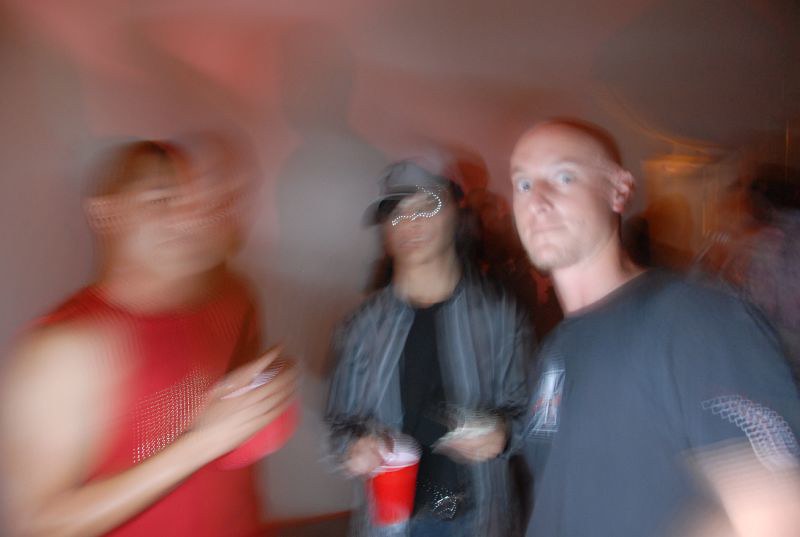A blurry photograph captures a dynamic moment with at least three identifiable individuals, possibly in motion. The primary figures include three men, all seemingly focused on the camera. On the left, a man wears a red, sleeveless shirt. In the center, another man is dressed in a gray shirt over a black t-shirt, accessorized with a belt, hat, and glasses. He has longer hair and holds a red cup. The man on the right, the most clearly visible, wears a gray shirt, is bald, and also holds a red cup, staring intently at the camera. There appears to be a fourth person in the background, partially visible. The backdrop is a plain white wall, casting shadows from the figures in the scene.